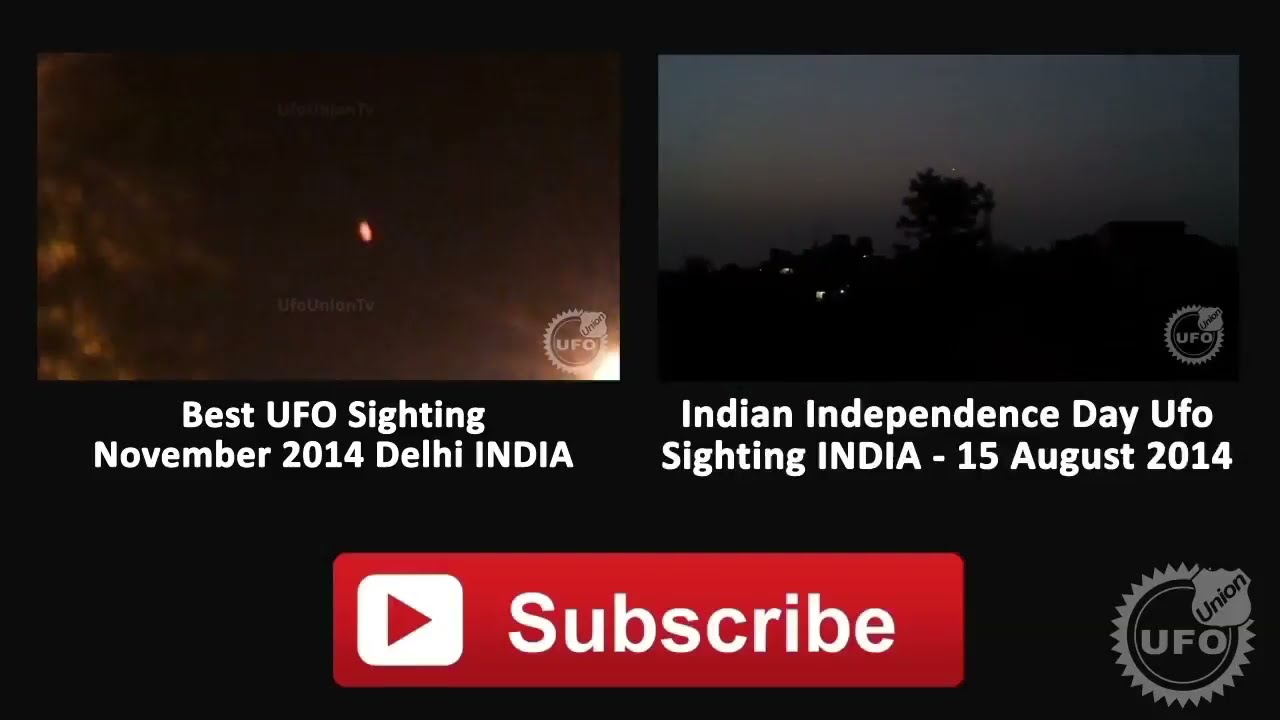The image is a screenshot from the end of a YouTube video, showcasing two suggested videos from the same channel, UFO Union. At the bottom of the screen, there is a large red subscribe button next to the channel's gear-logo with the text "UFO Union." The left video thumbnail features a grainy, sepia-toned nighttime scene with a yellow spot in the sky, titled "Best UFO Sighting November 2014 Delhi, India." The right thumbnail shows silhouettes of trees against an illuminated sky with city lights and is labeled "Indian Independence Day UFO Sighting India 15th August 2014." The predominant colors in the image are red, white, gray, black, and blue. Overall, the image strongly encourages viewers to subscribe to the channel after viewing the two dramatic UFO sighting videos.